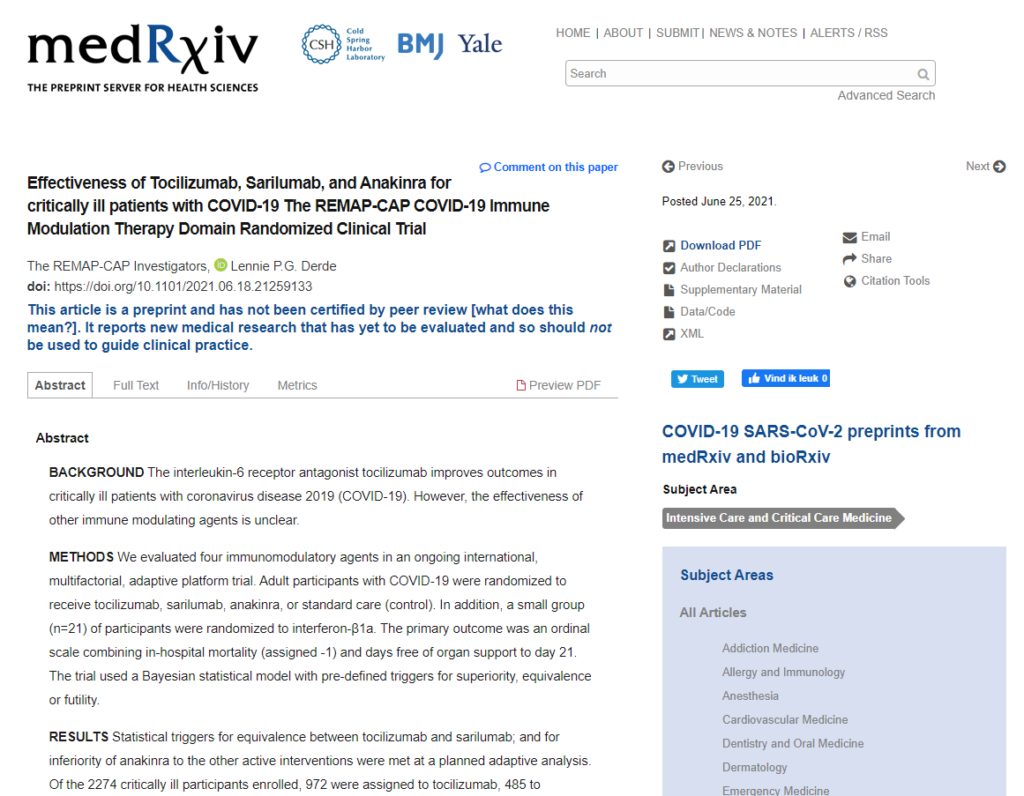The image titled "MedRxiv" features a snapshot of the preprint server specifically dedicated to health sciences. The MedRxiv platform prominently displays its association with CSH, BMJ, and Yale. At the top of the interface, there is a navigation bar that includes options such as Home, About, Submit, News and Notes, Alerts, and RSS. 

Central to the image is a search bar, with a highlighted section below mentioning "Effectiveness of" antibiotics for critically ill COVID-19 patients. This is a part of the REMAP-CAP COVID-19 Immune Modulation Therapy Domain Randomized Clinical Trial, targeting COVID-19 through clinical trials. The image includes a portion where users are prompted to comment on the paper, presented in blue text. There are navigation buttons labeled Previous and Next, and a posting date of June 25th, 2021. Additionally, there is an option to download the PDF of the document.

Further down, the image references various functionalities and sections such as Other Categories, Email, Share, Author Declaration, and Supplementary Material. It mentions a disclaimer that the article is a preprint and has not undergone peer review, indicating that it conveys new medical research that should not be used to guide clinical practice until evaluated.

The image outlines sections like Abstract (enclosed in a box), Full Text, Info/History, and Metrics. The Abstract section is subdivided into Background, Methods, and Results, each accompanied by a descriptive write-up.

On the right-hand side of the image, there is a section dedicated to COVID-19 and SARS preprints, along with options to view all articles under various subject areas.